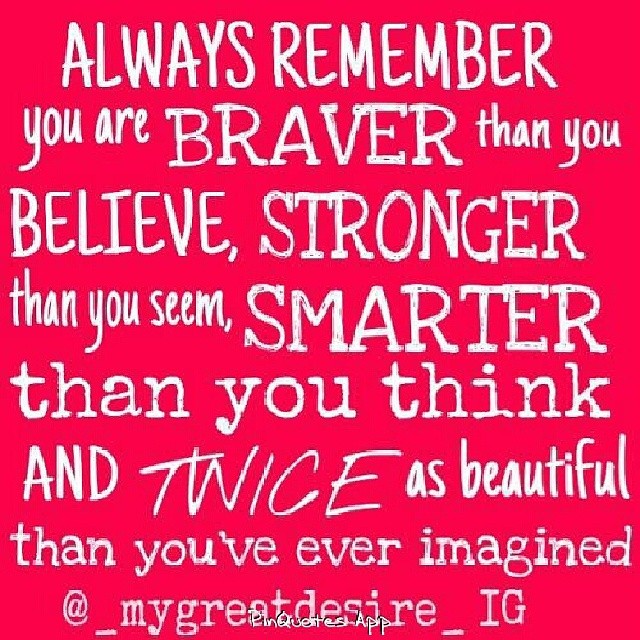This meme image features a bright red square background with white text that delivers a motivational message. The text reads, "Always remember you are braver than you believe, stronger than you seem, smarter than you think, and twice as beautiful than you ever imagined." The typography is a blend of various fonts, showcasing a mix of uppercase and lowercase letters, with the word "twice" uniquely italicized. Some fonts are bold and thick, while others are thin or resemble script and typewriter styles. The image appears to be a cropped screenshot, finished off with an Instagram handle at the bottom, written as @ _my great desire_, followed by the letters IG, which stand for Instagram.